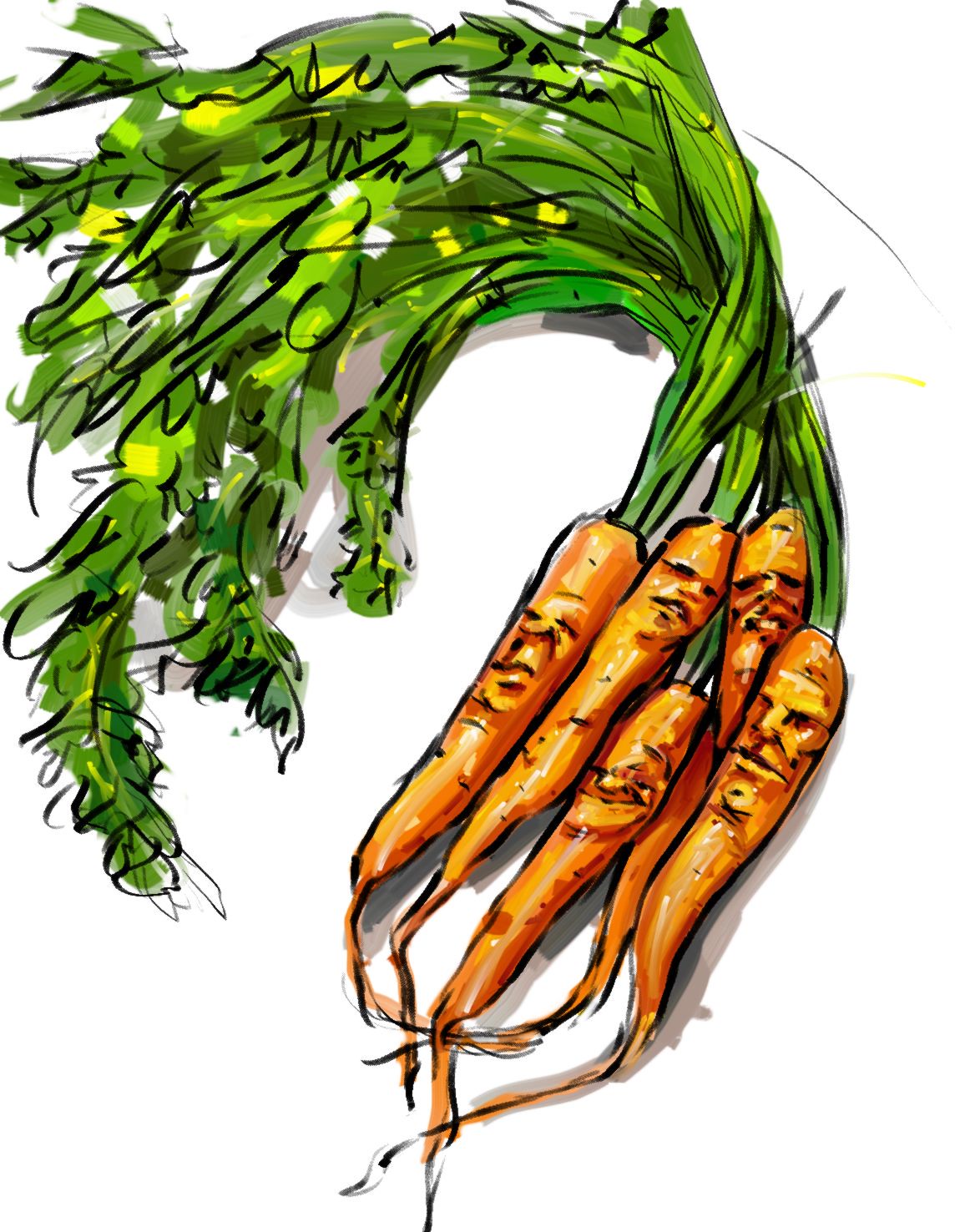This image is a detailed, cute cartoon-style drawing of five to six carrots on a white background. Rendered with a technique resembling colored markers, the carrots are depicted in lovely shades of bright orange contrasted with white highlights and dark outlines. Each carrot has distinct, subtly grim faces carved or drawn on them, featuring closed eyes, noses, and mouths. The green leafy tops of the carrots, rich with varying shades of green and yellow and accented with black squiggles, swoop up and away, curling to the left and sometimes reaching back down almost to the carrot bottoms, which show fine roots with black lines. The scene includes subtle gray shadows, adding depth and contrast to the whimsical arrangement of these anthropomorphic vegetables.